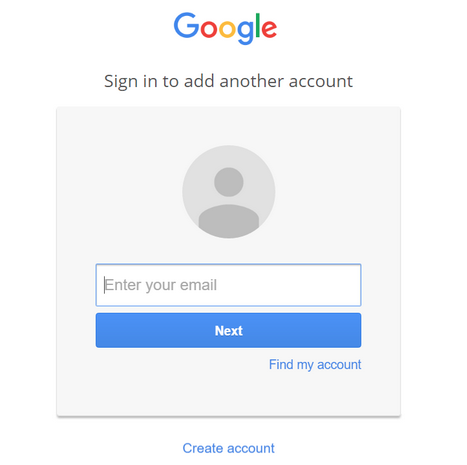The image is a screenshot of the Google sign-in page. At the top, the recognizable Google logo is displayed in its usual multi-colored letters: the "G" in blue, the first "O" and the "E" in red, the middle "O" in yellow, and the "L" and "E" in green. Below the logo, the text reads "Sign in to add another account."

The central portion of the screenshot features a light gray square with a person icon placeholder representing the profile picture. Below this icon is a white input field with a blinking cursor, accompanied by the prompt "Enter your email."

Beneath the input field, there is a blue rectangular button with "Next" written in white. This button is prominently placed for users to proceed after entering their email. Below this button, the text "Find my account" is displayed in blue, not enclosed in a button, offering another option. At the bottom of the gray square, "Create account" is also written in blue, inviting new users to register.

The entire interface sits against a simple white background, suggesting a clean and uncluttered design. While the dimensions and proportions hint that this might be a screenshot from a mobile device—appearing taller than it is wide—it could also be a capture from a computer screen. The absence of other screen elements makes it difficult to be certain.